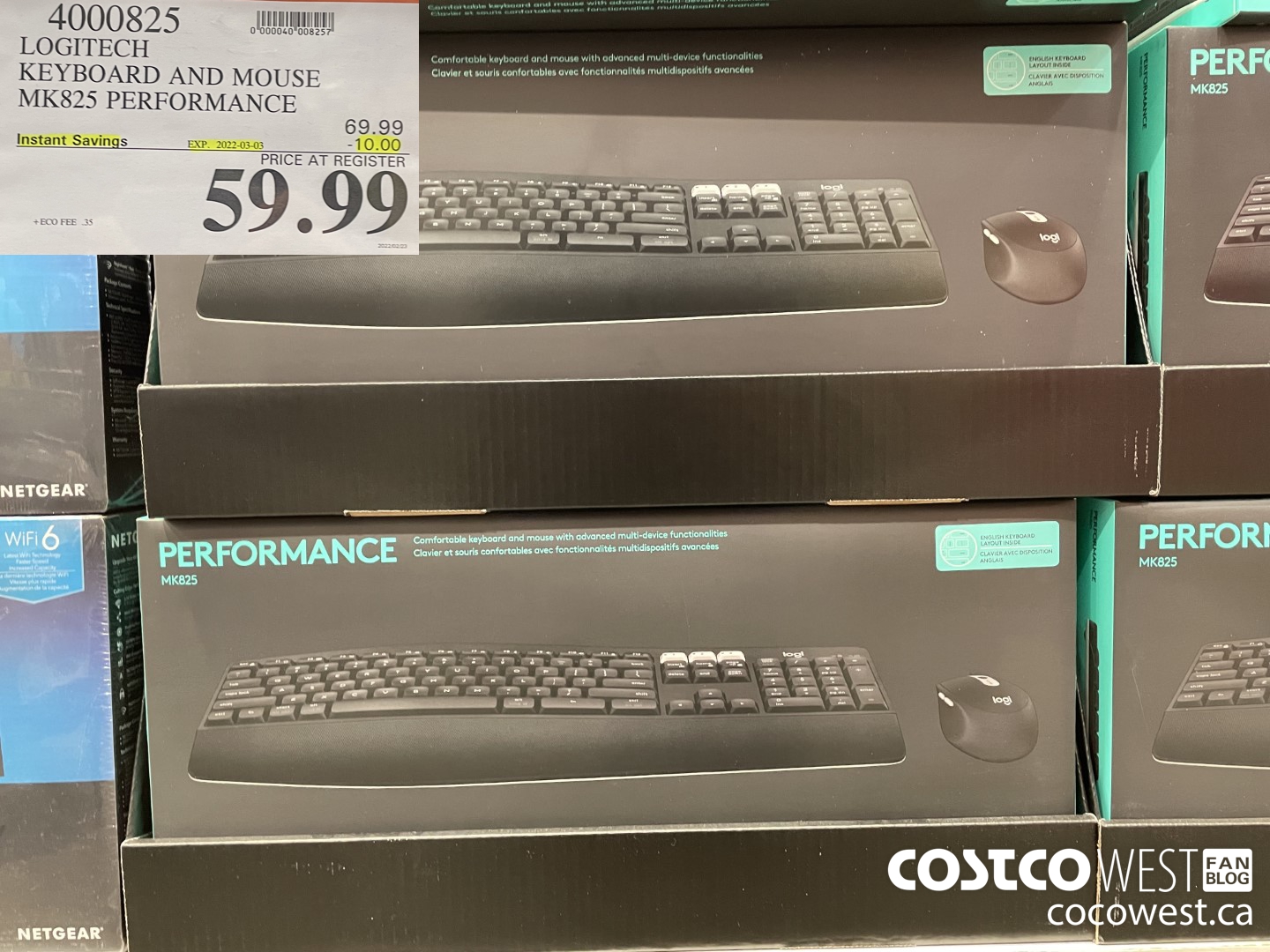This image appears to be a screenshot from a website, evident from the text "Costco West" and the URL "CoCoWest.ca" displayed in white at the bottom right corner. The photograph features a close-up view of several boxed computer keyboards on display in a store. Two prominent boxes in the center are branded Logitech, identifiable by their grayish color and detailed illustrations of the external keyboards and mice they contain. The mouse is depicted on the right side of each box. In the upper left corner of the image, there's a white shelf label displaying the item number 400825. Below this number, in capital letters, it reads "Logitech Keyboard and Mouse MK825 Performance." The price, "59.99," is prominently shown in large black numbers at the lower right corner of the label.